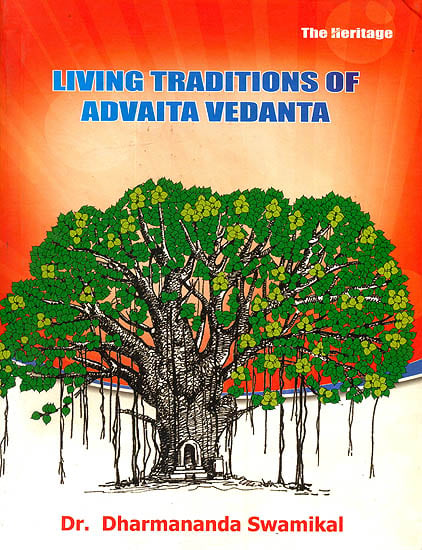The image appears to be a scan of a magazine cover, possibly "The Heritage," depicting a detailed drawing in a portrait layout. The top half of the image features an orange background with white and blue text. In the upper right corner, white text reads "The Heritage," while centered at the top in blue text outlined in white is the title "Living Traditions of Advaita Vedanta." Below this, the background transitions to a white backdrop that highlights a prominent tree. 

The tree has a black trunk and base, and features both dark and light green leaves. Hanging from its branches are what appears to be strands similar to Spanish moss. The trunk has distinctive black and white striped patterns and houses a small archway at its base, resembling a doorway with steps leading up to it. Beneath the tree, on the white background, is the name "Dr. Dharmananda Swamikal" in orange text.

Overall, the image combines vibrant colors and intricate details to emphasize the significance of the tree and the associated text, presenting a harmonious blend of traditional and stylized elements.